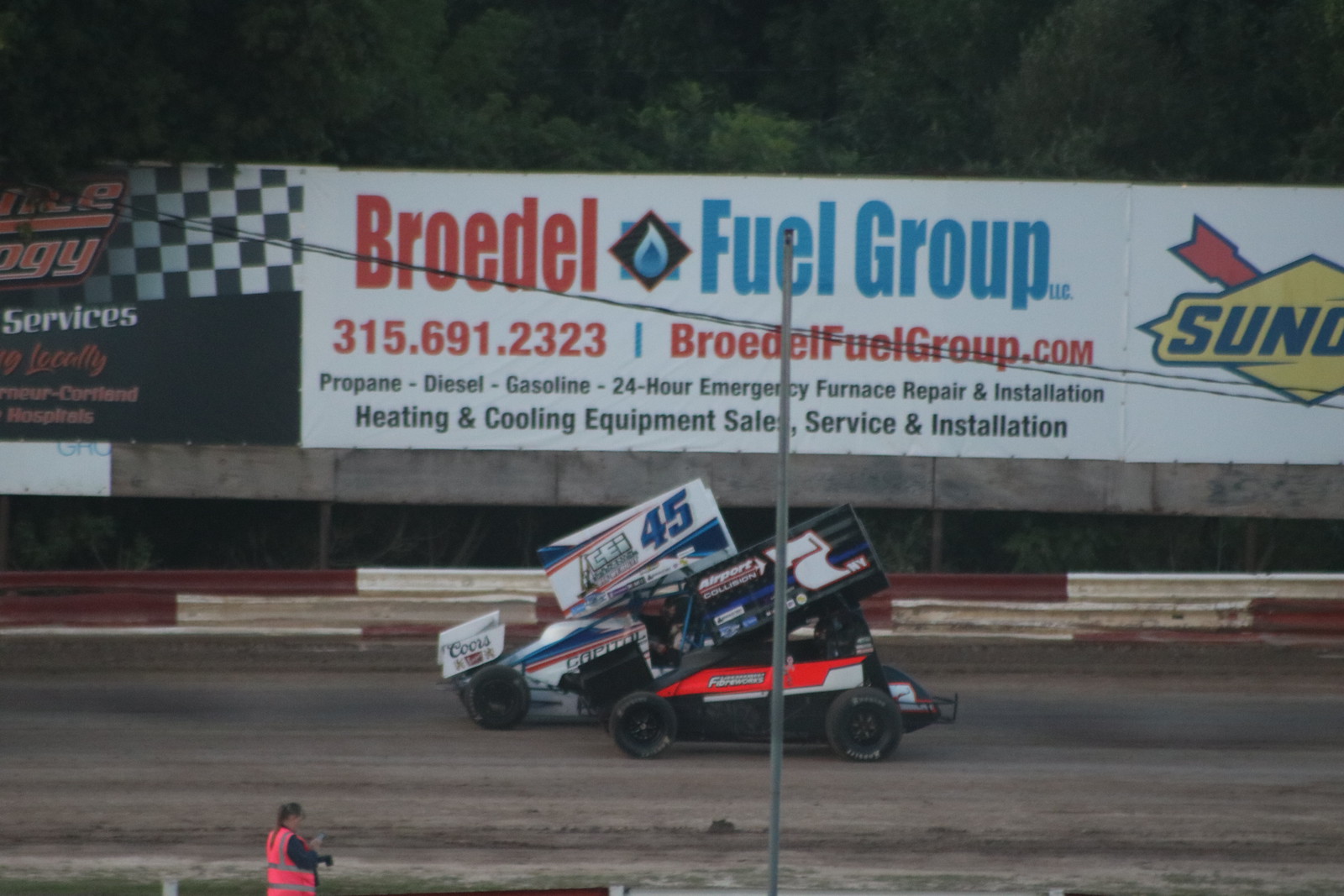The image captures a dynamic scene on a dirt racetrack with two specialized race cars. The car closest to the camera features a striking orange panel on its black body, accentuated by black tires and a prominent fin adorned with advertisements in white text on a black background. To its left, another race car, predominantly white, displays the number 45 in blue on its spoiler and the "Coors Light" symbol above its front tires. Both vehicles sport large, distinctive wings atop their roofs, giving them a toy-like appearance. In the background, a vivid banner reads "Broaddale Fuel Group" against a white backdrop, alongside a blue square graphic and comprehensive service details. Adjacent is a partially visible Sunoco logo on a yellow background, characterized by an orange arrow. On the far edge of the track, a woman in a pink safety vest stands near a red and white barrier. The scene also includes a patch of green on the bottom left and a backdrop of green trees, further adding to the vibrant, detailed setting.